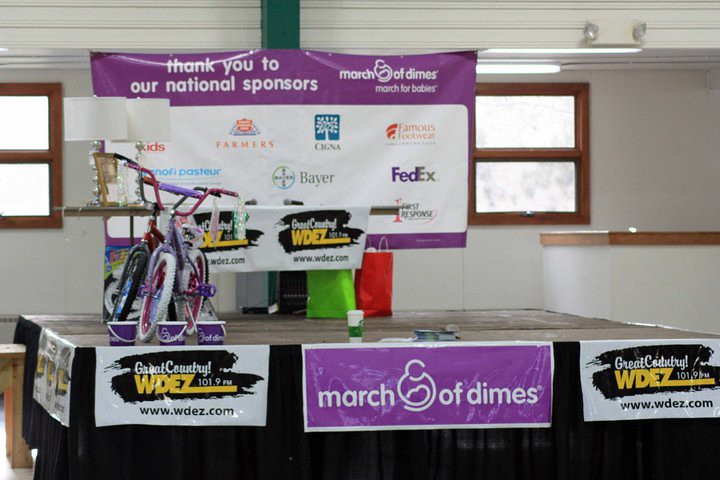This color photograph captures a detailed scene of a small stage area inside a room, decorated for a March of Dimes event. The stage features two children's bicycles—one with white tires and the other with black tires—positioned on the left. Scattered around the stage are multiple purple buckets and a Starbucks coffee cup. Banners adorn the stage, prominently including a purple March of Dimes banner at the front and various sponsor banners such as WDEZ 101.9 FM. The backdrop also features a large purple banner with the March of Dimes logo, listing national sponsors like FedEx, Farmers Insurance, Bayer, and Cigna. The stage is surrounded by a black curtain, and behind it, a couple of closed windows can be seen on the wall. The overall display emphasizes the collaboration and sponsorship for the event, celebrating support from various organizations.